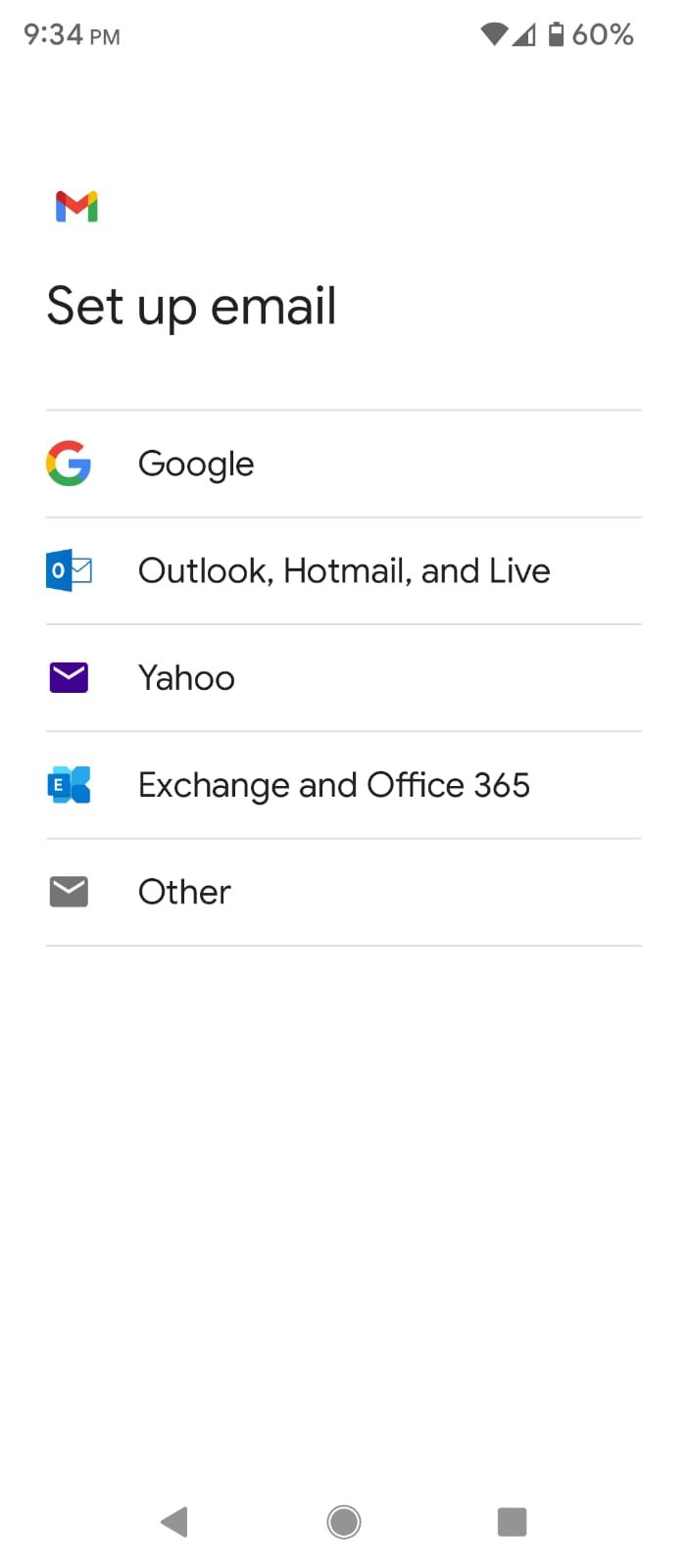This image is a screenshot from a cell phone, captured at 9:34 PM. In the upper right-hand corner of the screen, several icons are visible, including a fully connected Wi-Fi signal, a cell phone reception icon showing three out of four bars, and a battery icon indicating 60% remaining charge. To the right of these icons is the Google Mail logo, represented by an "M."

The main portion of the screenshot displays a setup interface for configuring email accounts. Large black text reads "Set Up Email," separated by a gray horizontal line. Below this, there are five options for email configuration, each with its corresponding logo to the left:

1. **Google** - accompanied by the distinctive "G" logo
2. **Outlook, Hotmail, and Live** - featuring the Outlook envelope icon
3. **Yahoo** - marked by the purple envelope icon
4. **Exchange and Office 365** - no specific icon is mentioned
5. **Other** - no specific icon is mentioned

This screenshot is likely from an initial setup or settings menu on a smartphone, guiding the user through the process of adding an email account.